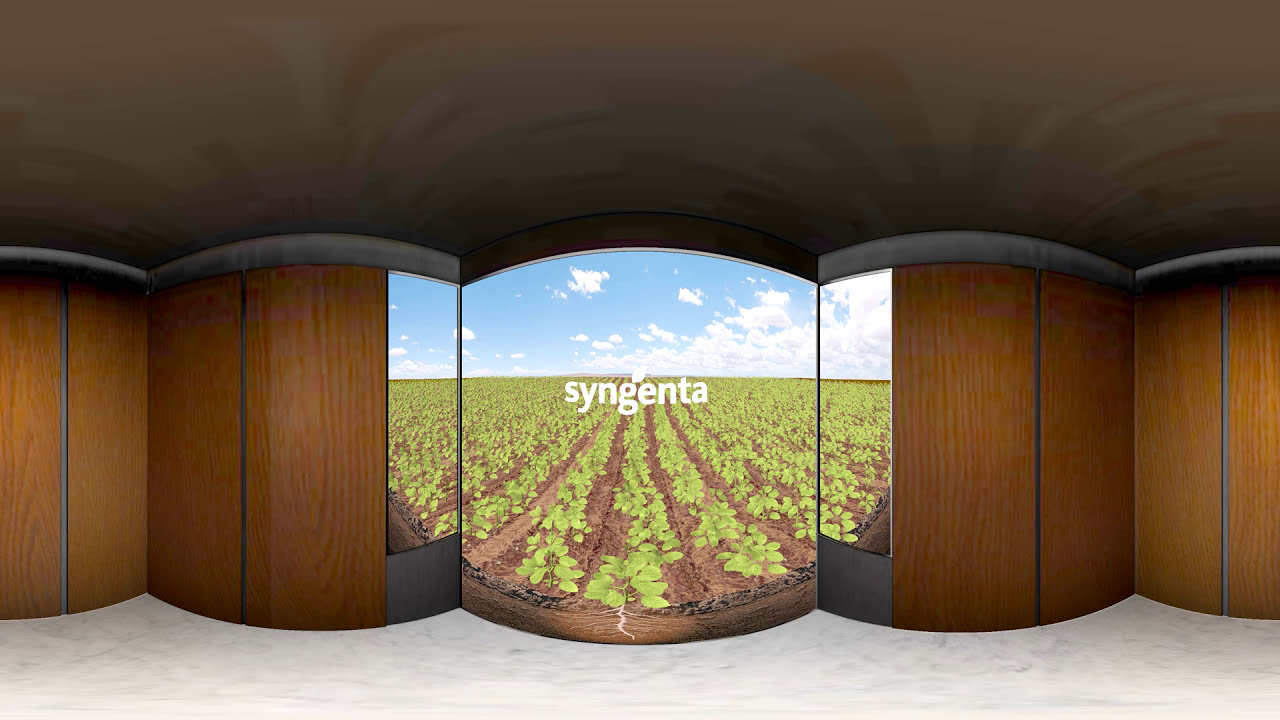The image presents a computer-generated, panoramic view inside a uniquely designed room with distinctive architecture. The setting appears to be a small, indoor space characterized by curved, wooden paneled walls that bulge outward and inward intermittently. Central to the image is a striking feature—a set of three convex screens seamlessly integrated into the wooden wall, displaying an expansive, digitally rendered farmland scene. Rows of low-growing, leafy green crops stretch out under a blue sky dotted with puffy white clouds, suggesting a sunny day. Prominently displayed at the horizon within this simulated landscape is the brand name "Syngenta" in white lowercase letters. The room's floor is a pristine white, possibly marble, while the ceiling is dark gray with various textures, adding to the intricate design. The overall clarity and the highly polished nature of the image suggest it is intended for a virtual reality or augmented reality simulation, providing a hyper-realistic yet unmistakably synthetic environment.